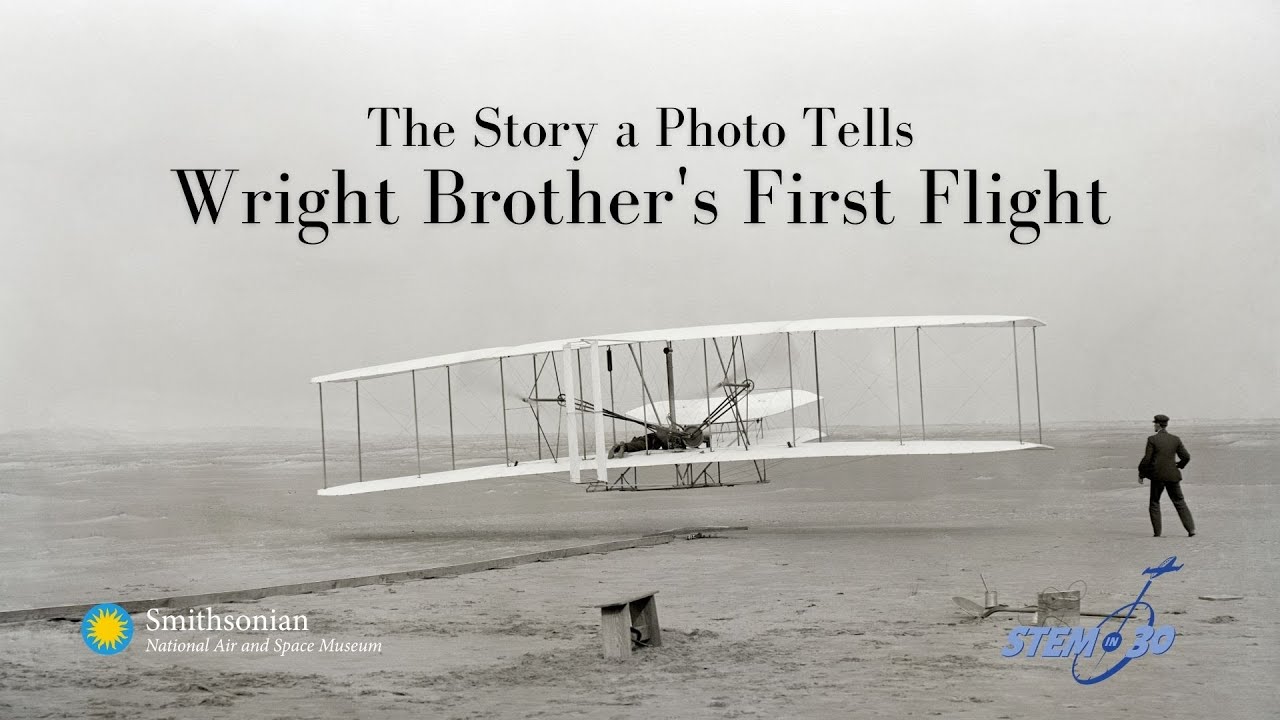In this black and white photograph, we see the historic Wright Brothers' first flight plane, a white biplane, positioned on a dirt field. The plane's structural details are evident, with two sets of horizontal wings interconnected by vertical black posts. In the background, a grayish sky looms overhead, contrasting with the monochrome ground. The scene includes a man dressed in a black suit and hat, standing to the right of the plane with his back to the camera, one foot positioned slightly forward. 

Overlaying the image are several pieces of text and logos. Centered at the top, in black letters, it reads: "The story a photo tells: Wright Brothers' first flight." To the far left, the Smithsonian National Air and Space Museum is credited, accompanied by a blue circular logo featuring a yellow sun. At the bottom right corner, there is another blue logo with the text "STEM" followed by the number "30," depicting a plane ascending from the top of a circle. The gray-white sky occupies the majority of the upper portion of the image, and a small wooden bench is visible in the foreground on the sandy terrain, adding historical context to the photograph.